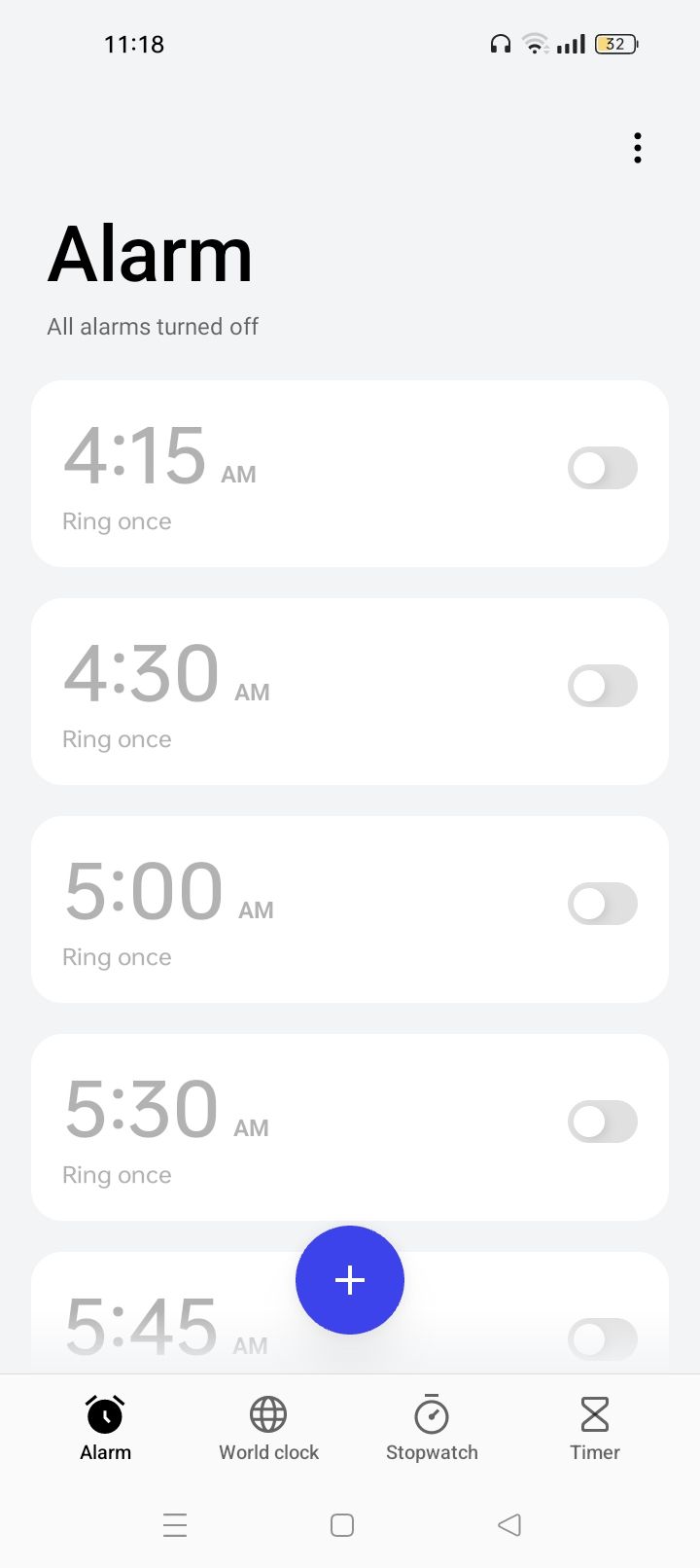This screenshot captures the alarm settings screen of a mobile phone. The background color is a light gray, and the status bar at the top displays the current time, "1:18," in the top left corner. In the top right corner, a battery percentage of "52%" is shown alongside a battery icon, indicating that headphones are connected.

At the very top of the screen, the word "ALARM" is prominently displayed in black letters. Below that, in smaller black letters, the text "ALL ALARMS TURNED OFF" confirms that no alarms are currently activated.

The main section of the screen contains five distinct sections, each with a white background and a toggle switch on the right side. Each section represents a different alarm time:

1. The first alarm is set for 4:15 AM, labeled "RING ONCE," and its toggle switch is off.
2. The second alarm is set for 4:30 AM, labeled "RING ONCE," and its toggle switch is off.
3. The third alarm is set for 5:00 AM, labeled "RING ONCE," and its toggle switch is off.
4. The fourth alarm is set for 5:15 AM, labeled "RING ONCE," and its toggle switch is off.
5. The fifth alarm is set for 5:30 AM, labeled "RING ONCE," and its toggle switch is off.

At the bottom center of the screen, there is a blue circular button featuring a white plus sign, suggesting an option to add a new alarm.